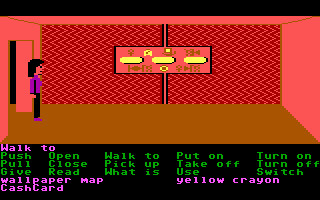Screenshot of a retro-style 2D video game. The scene depicts a character standing in a vibrant room with distinct design elements. The floor is a warm brown color, while the side walls are painted pink. The back wall features a striking chevron pattern with alternating red and pink stripes, adding a dynamic visual appeal. In the center of the scene, there is a noticeable sign whose details are unclear. The character, resembling a classic video game avatar, is wearing a purple shirt and black pants, and is positioned in front of a doorway located to the left side of the room. At the bottom of the screen, a black interface displays various action options in purple and green text, including commands like "walk to," "push open," "pull close," "put on," "turn on," "switch," "wallpaper," and "map," among others.